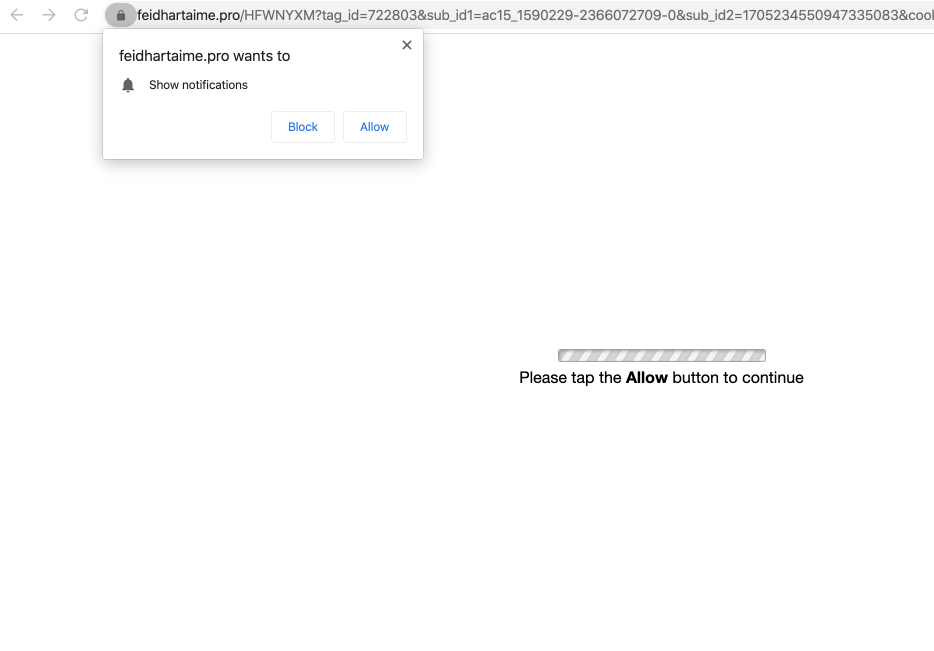The screenshot depicts a webpage belonging to the site "fidehartame.pro," with a pop-up notification that states, "This site wants to show notifications." Users are given the options to "Allow" or "Block" these notifications. The main content of the page is sparse, dominated by a white background. Centrally located is a message prompting users to "please tap the allow button to continue," suggesting that enabling notifications is necessary to access the site's functionality. Above this message is a small, horizontally striped status bar in white and gray, mimicking a loading or processing indicator. The image seems to be captured in Google Chrome, although most of the browser interface is cropped out.